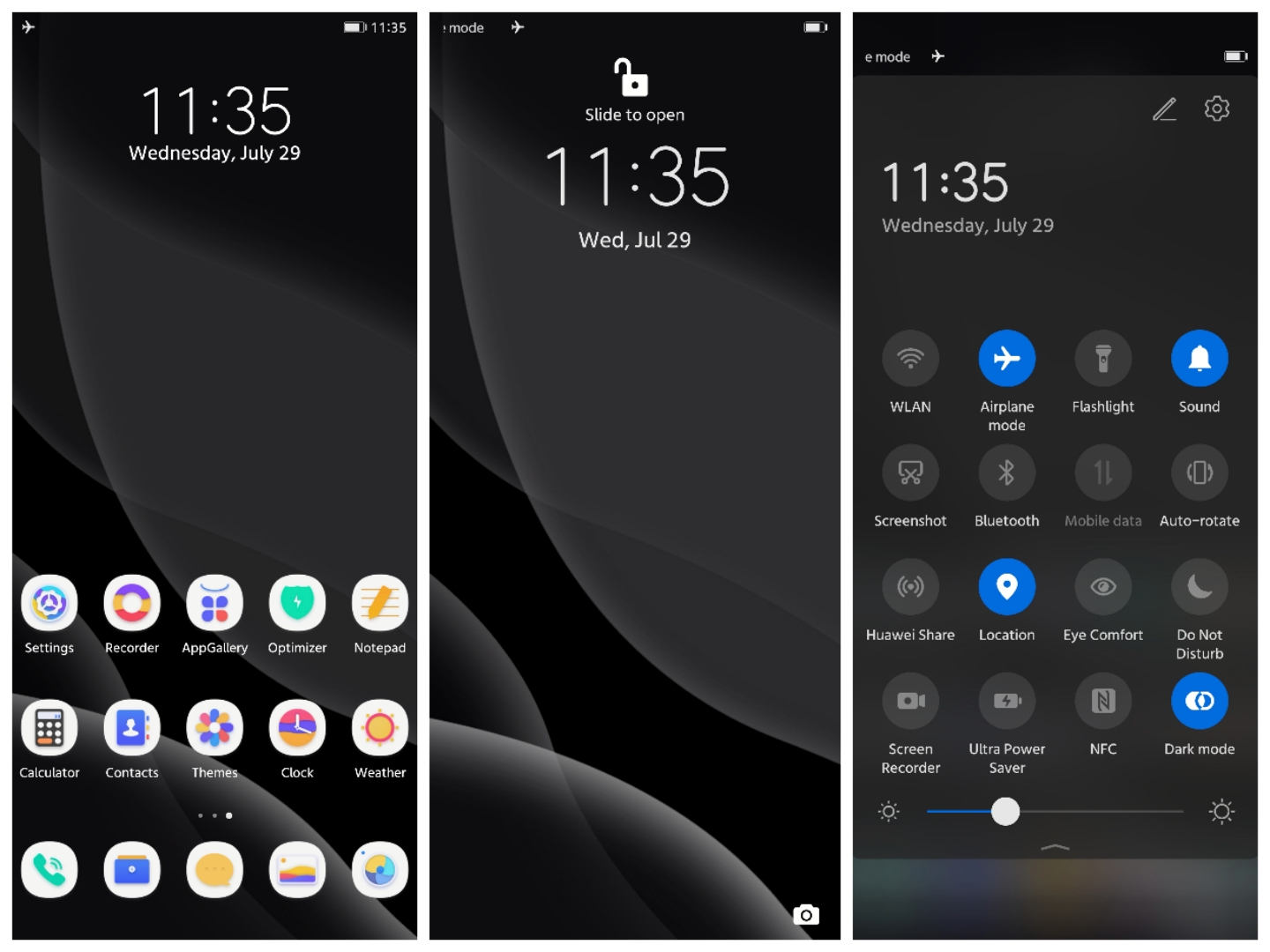Three sequential screenshots from a smartphone display the device's state and various screens at 11:35 AM on Wednesday, July 29th, with airplane mode activated. 

In the first screenshot, the home screen is visible, showcasing a nearly full battery. The array of installed apps includes Settings, Recorder, App Gallery, Optimizer, Notepad, Calculator, Contacts, Themes, Clock, and Weather. At the bottom, five additional apps are partially identified, with icons suggesting Phone and possibly Photos among them.

The second screenshot captures the lock screen, showing the 'Slide to open' prompt, maintaining the same date and time, with airplane mode still on. A small camera icon is positioned at the bottom right corner for quick access to the camera function.

The final screenshot delves into the Settings menu, still timestamped at 11:35 AM on the same date. Detailed settings options are displayed, including Wi-Fi, Airplane mode, Flashlight, Sound, Screenshot, Bluetooth, Mobile Data, Auto Rotate, a sharing function, Location, Eye Comfort, Do Not Disturb, Screen Recorder, Ultra Power Saver, NFC, and Dark Mode. The screen also features a brightness customization slider for adjusting the display's backlight intensity.